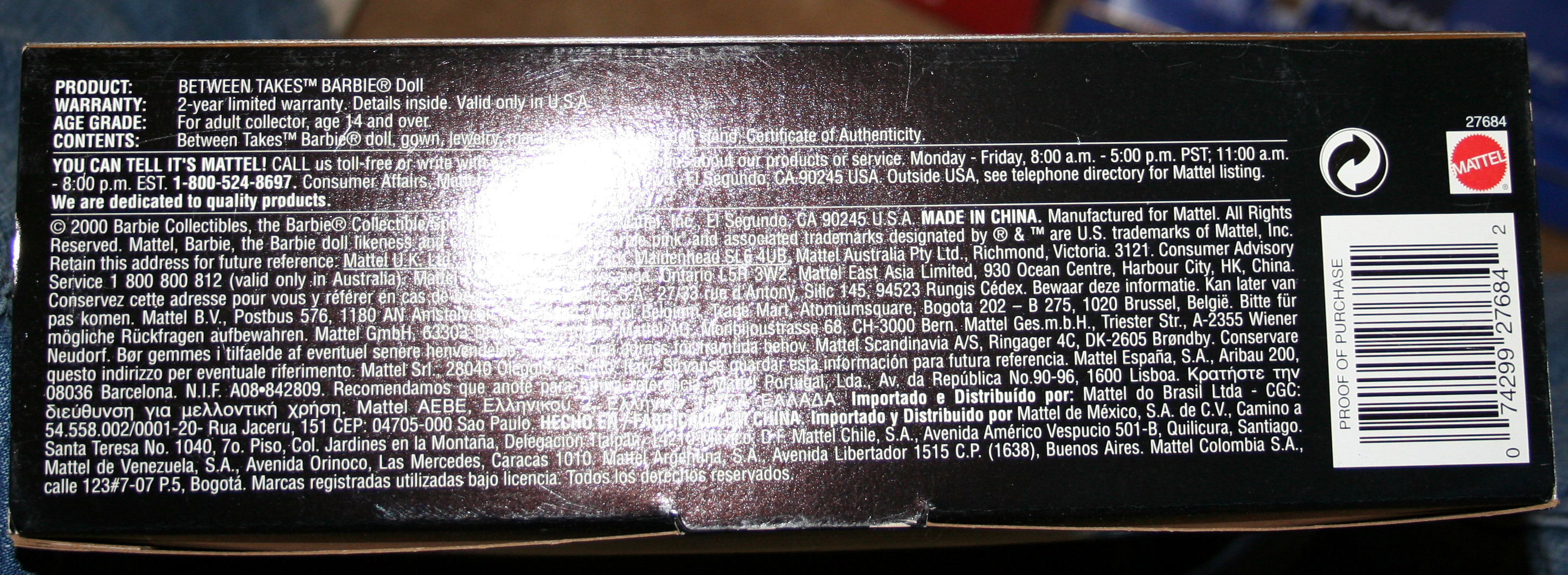This image shows a detailed close-up of a product label featuring reflective, shiny paper and a visible glare from a camera flash, which obscures part of the text. The label is primarily brown and seems to list product information in various languages, though much of it is illegible due to the glare. 

At the top of the label, the readable text clearly states: "Product: Between Takes Barbie Doll. Warranty: Two-year limited. Details inside. Valid only in US. Age grade: For adult collector, age 14 and over." The label also lists the contents of the box as a "Between Takes Barbie Doll, gown, and jewelry."

The brand information is present, indicating it is a Mattel product. This is confirmed by a toll-free number and a commitment to quality from Mattel. The label continues with about 10 to 12 lines of very small print, likely listing further product details and warranty information in multiple languages.

To the right of this text block, there's a recycle symbol, the Mattel logo—distinguished by a red circular design with a white square and the word "Mattel" in white—and finally, a barcode with "Proof of Purchase" written above it.